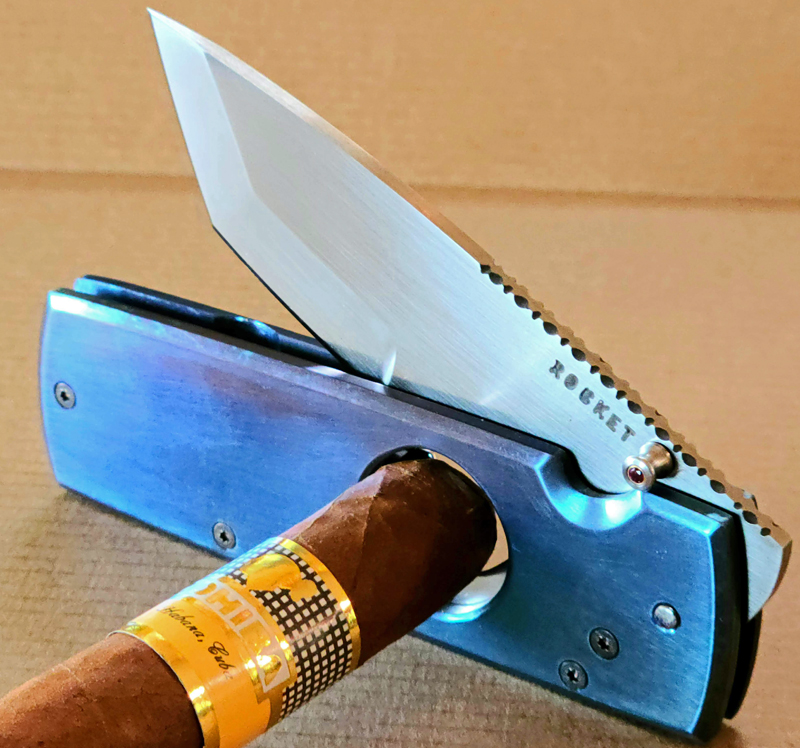The image depicts a close-up of a cigar being cut by a specialized utility knife that also functions as a cigar cutter. The cigar, featuring a yellow label adorned with black and white designs, has text in white and cursive black font along with a gold edge around the wrapper. This brown cigar is positioned within the cutter's central hole. The utility knife has a metallic blue body with four visible screws and a polished silver blade that has "ROCKET" engraved on its top right. The knife blade is partially open, prepared to slice through the cigar, and the surrounding environment is lit brightly with a clear, light brown background.